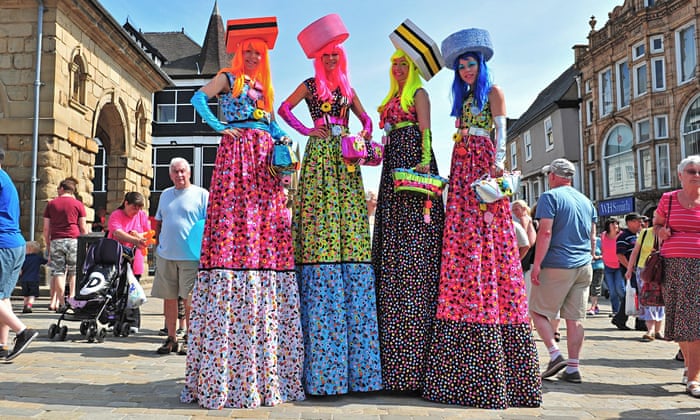In the middle of a bustling street scene with stone buildings featuring arched windows and doorways, four exceptionally tall women appear to tower above regular pedestrians, likely perched on concealed stilts. They wear eclectic, avant-garde outfits accentuated by neon wigs and dramatic hats, making an impression akin to a fashion event. 

From left to right:
- The first woman sports an orange wig and a square orange hat with a black center, smiling directly at the camera. She wears blue fingerless gloves stretching to her elbows and a dress with a blue top, a pink middle, and a white bottom, all adorned with polka dots.
- The second woman is under a circular pink hat and has a hot pink wig. She also smiles at the camera, wearing pink fingerless gloves and a dress comprising a black top, followed by green and blue sections, also decorated with polka dots.
- The third woman, looking equally vibrant, has a neon green wig and a square hat in white, black, and yellow. She is donned in green fingerless gloves, a pink and black dress with a polka dot pattern, and holds a purse in her left hand.
- The fourth woman wears a circular blue hat and a matching blue wig. She smiles warmly while holding a silver purse in her left hand. Her dress consists of a yellow top followed by pink and black sections, continuing the polka dot theme, and she wears silver fingerless gloves extending past her elbows.

The colorful and whimsical nature of their attire contrasts sharply with the more subdued tones and historic architecture surrounding them. Passersby glance curiously at the tall, flamboyantly dressed women as they continue about their day.